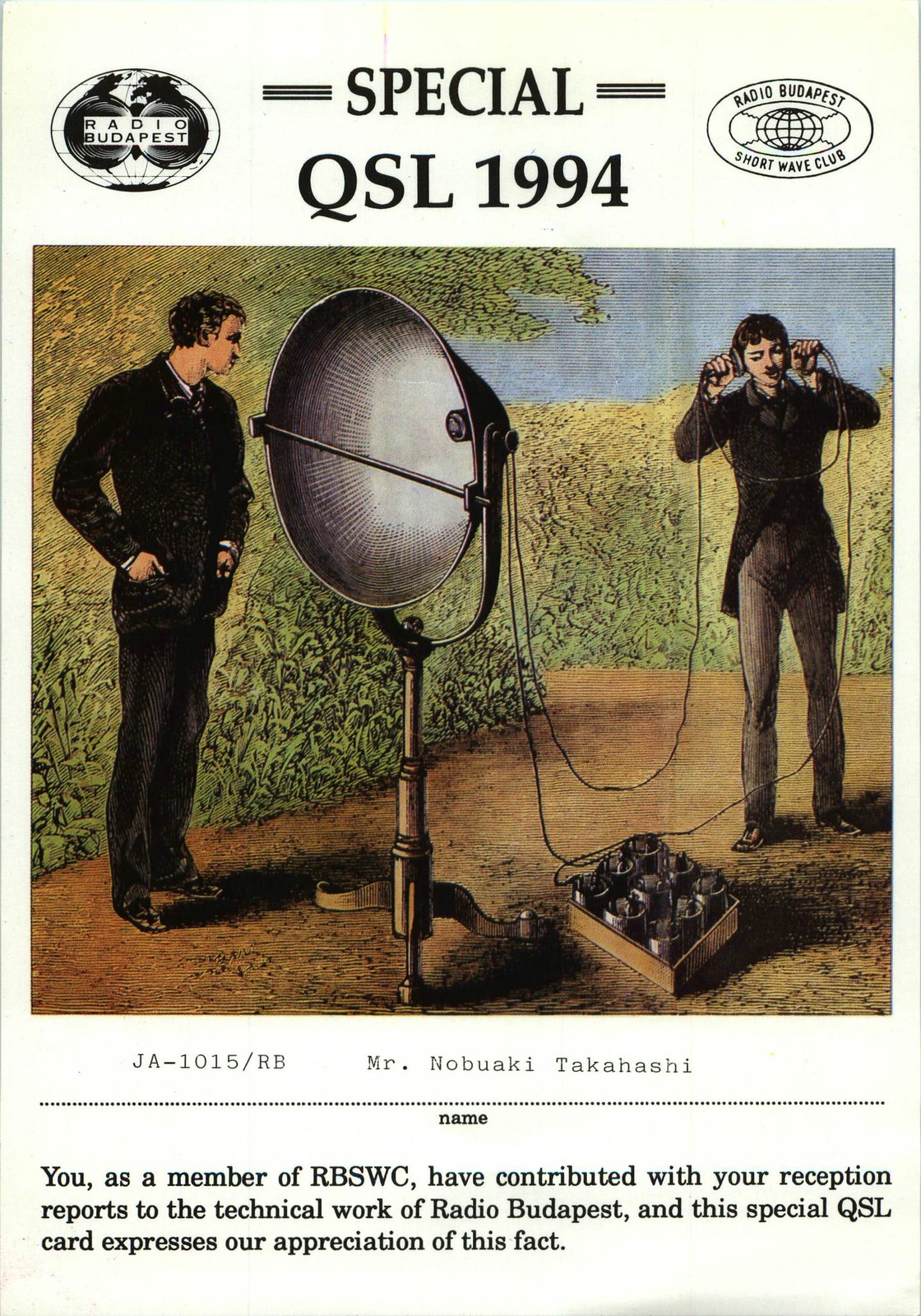The image is a colored printed pamphlet or program with a white background. In the upper left corner, it reads "Radio Budapest" with an illustration of the Earth. The title "Special QSL 1994" is prominently displayed with decorative lines on each side. On the right side, it features the text "Radio Budapest Shortwave Club" next to a circular logo. The main illustration shows two men: one wearing a black suit, and another with two ear pieces, akin to headphones, connected to a large radio antenna on a tripod. This scene is set against a backdrop featuring shrubs, a tree, a dirt road, and a blue sky. Below the image, a paragraph expresses appreciation to Mr. Nabuaki Takahashi and other members of the RBSWC (Radio Budapest Shortwave Club) for their reception reports, indicating they have contributed to the technical work of Radio Budapest. The paragraph reads: "You as a member of RBSWC have contributed with your reception reports to the technical work of Radio Budapest and this special QSL card expresses our appreciation of this fact."